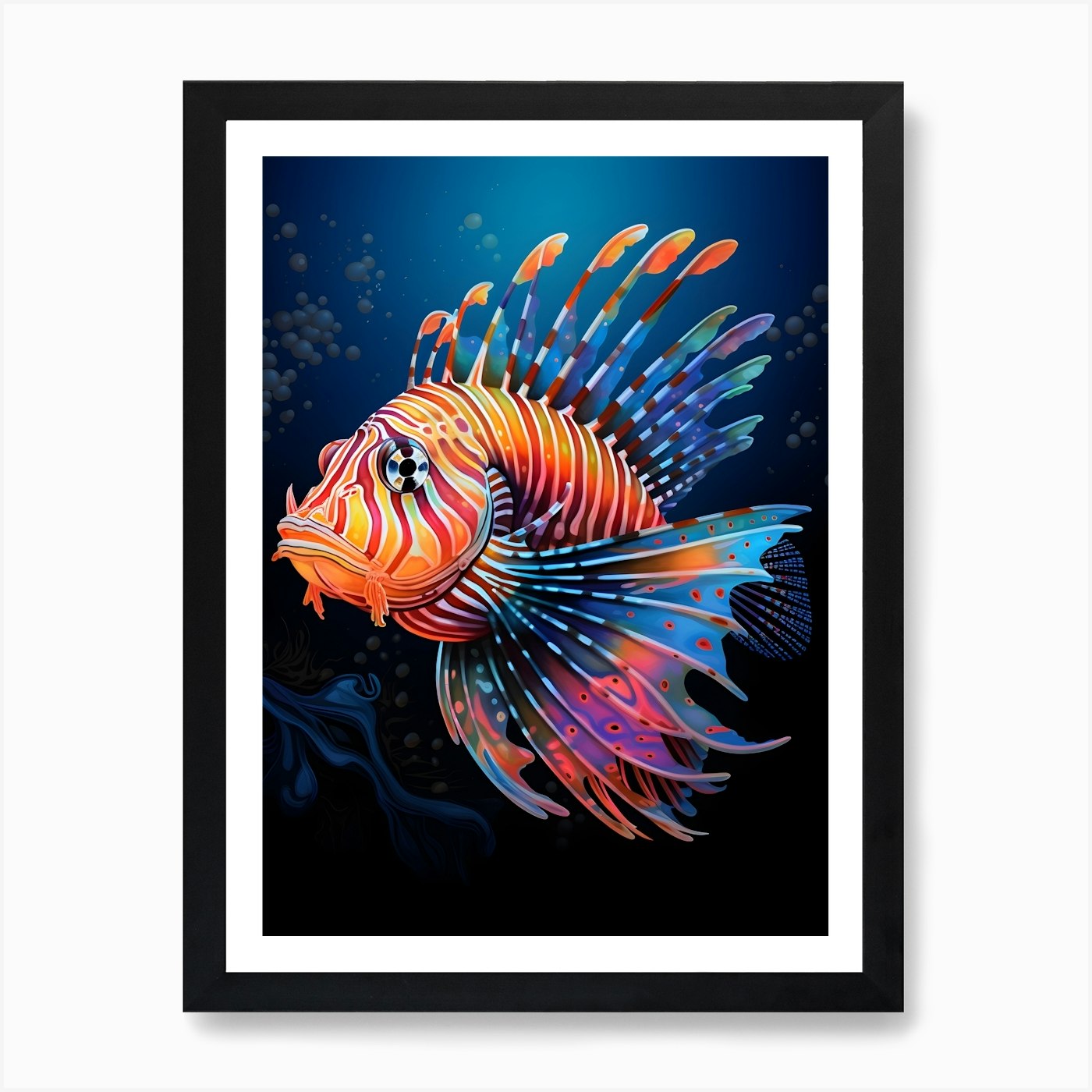This is a vibrant and detailed painting of a psychedelic, multi-colored fish encased in a black frame with a white matte border, set against a white surface. The underwater scene features a gradient background with medium blue water at the top transitioning to dark blue at the bottom, interspersed with bubbles on both the left and right sides. The fish, positioned to the left and facing left, boasts a dazzling array of colors: its face and head are adorned with orange, yellow, and red stripes, and it possesses a striking eye reminiscent of a CD with blue, black, and white hues. The gills on the left side of its body exhibit a palette of blue, orange, and blue with red spots, transitioning to pink. The fish's mouth is orange, and its back is striped in orange, red, and white, extending down to a dark blue tail. Its top spine fins resemble markers topped with feather-like extensions in light blue, brown, dark blue, and decorated with orange, purple, and blue colors. The overall impression is that of a fantastical, tropical underwater creature, enhanced by the swirling dark blue shapes and rising bubbles that complete the whimsical underwater ambiance.